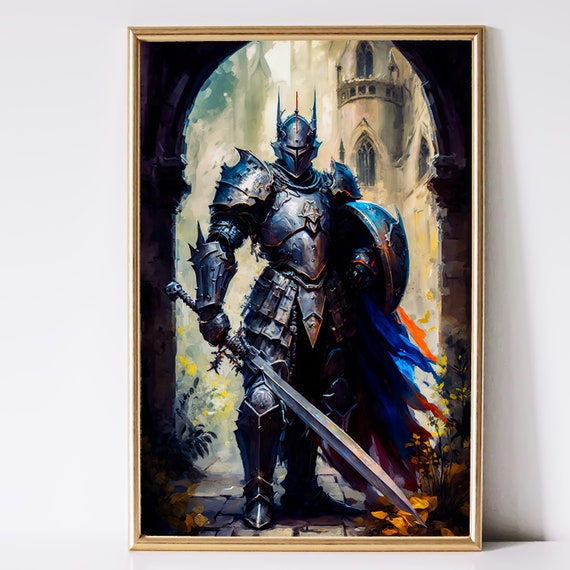This is a detailed painting set in a gold frame, which leans against a white wall, casting a slight shadow to the right. The central figure is a formidable knight clad in silver-gray, gleaming armor with prominent shoulder pads, thigh guards, and metallic boots. The closed helmet, featuring a narrow slit for the eyes and pointy ears, gives the knight an imposing presence. In his right hand, he brandishes a long sword with a silver blade and gray handle, while his left hand grips a round, gray shield. Flowing blue and orange fabrics, possibly part of a cape, drape from his armor. The knight stands resolutely in a stone archway, with a hint of a castle tower and a windowed balcony visible in the background. The base of the painting features leaves and rocky, brick elements, adding texture to the scene.